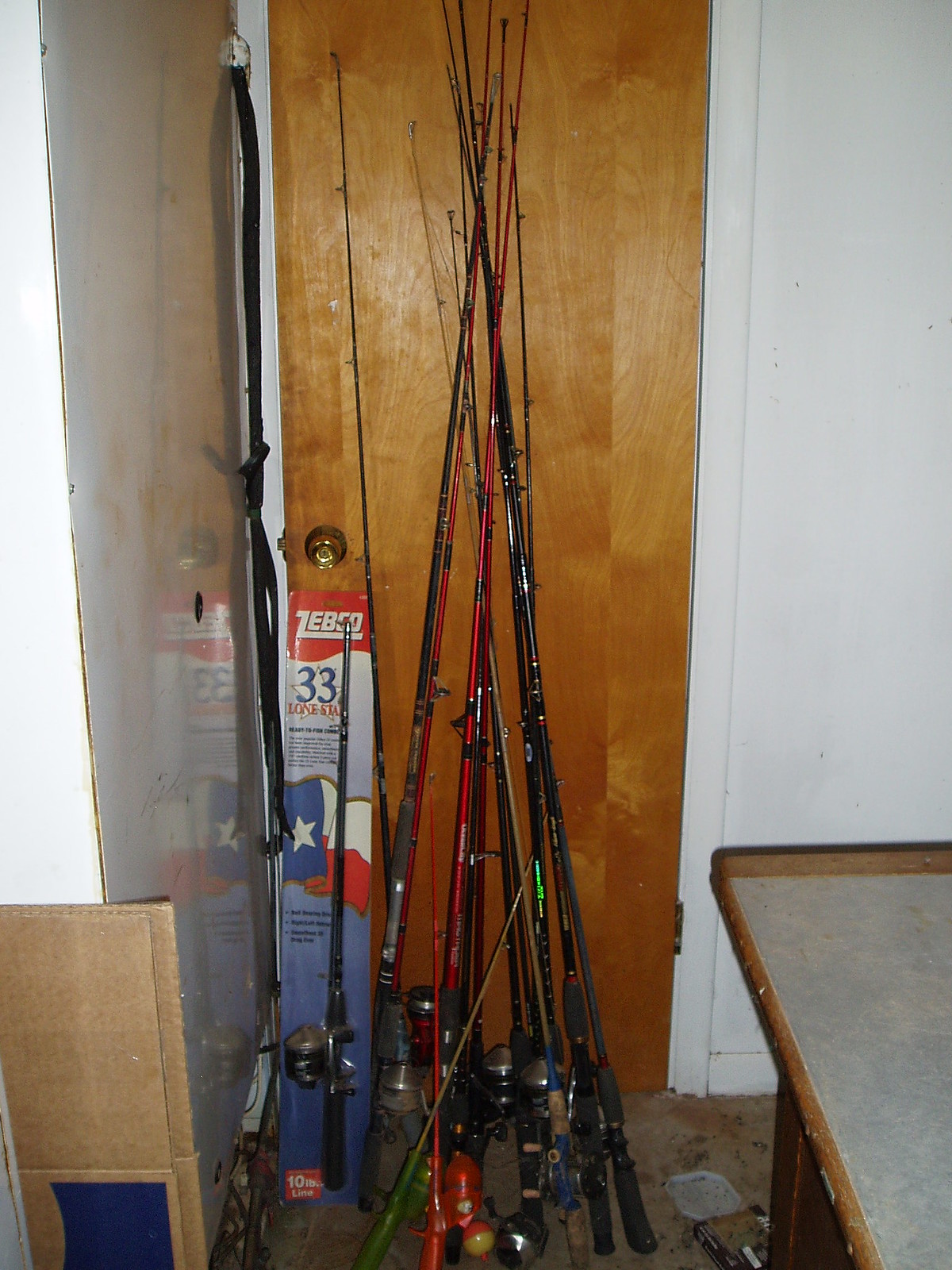The portrait-oriented color photograph prominently features a collection of fishing rods resting in a tipi-style arrangement against a mahogany-colored wooden door. The rods, varying in colors, sizes, and designs, have their handles positioned at the bottom, resting on the ground, and their tips crisscrossing at the top like the poles of a Native American tipi. Notably, one of the fishing rods is still in its original packaging, a Zebco 33-inch, with a distinct red, white, and blue label. The door they are leaning against is dark brown with visible wood grain, slightly ajar, equipped with a bronze round doorknob and a latch located halfway down on the left side. To the left of the door is a reflective white wall surface, likely the side of a cabinet. On the right of the rods is a table with a formica top. Additionally, a piece of black knotted rope extends from the ceiling. The composition of the image suggests an indoor setting, possibly a garage or utility room.